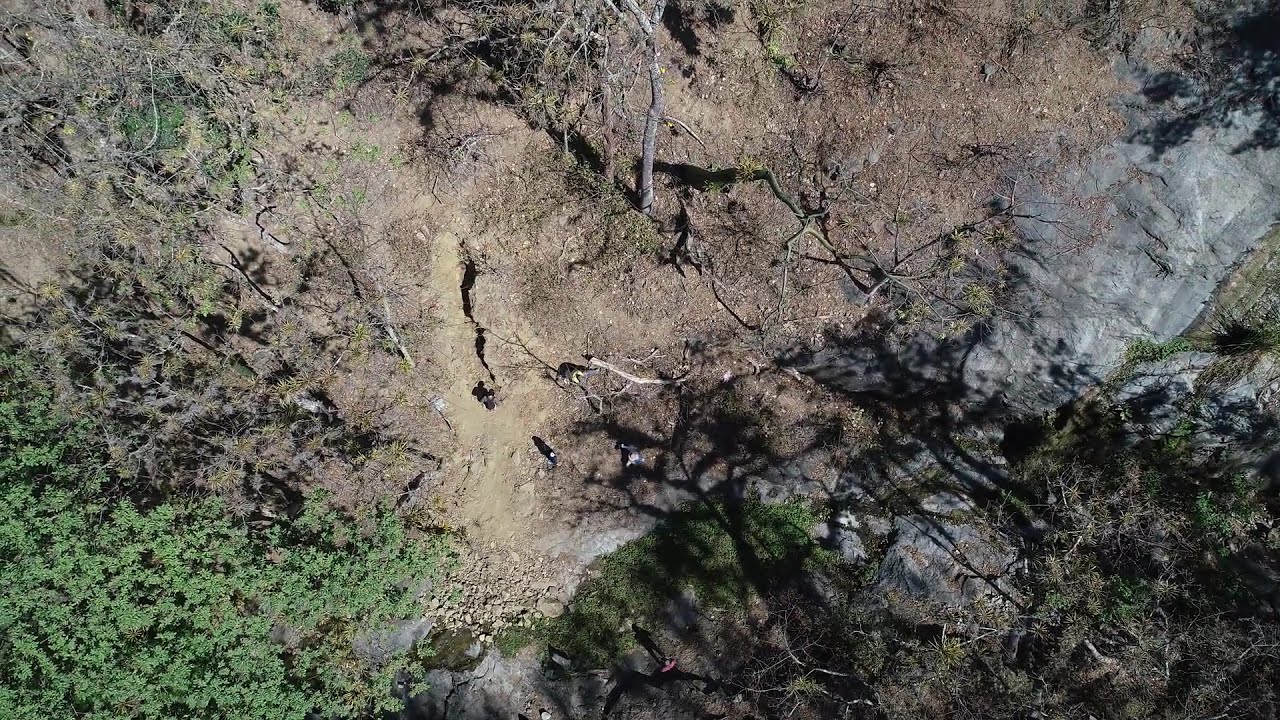This aerial photograph captures a barren, rocky landscape dominated by sandy brown earth interspersed with patches of green shrubs and the occasional tree. The overall environment is dry, resembling a desert with sparse vegetation, much of which appears yellowing or dead. In the lower left-hand corner, a vibrant green tree contrasts starkly with the otherwise desolate scene. To the upper right, the terrain transitions into a large expanse of flat gray rock peppered with some green moss or low-growing plants. Scattered throughout the image are what seem to be human figures; three or possibly four are standing at the vertices of what looks like a square formation, with one figure positioned at the top of a ravine. The lower right-hand corner reveals a chaotic mix of dead brambles and brush, and between some large gray rocks, there might be another person partially obscured. This aerial view, possibly of a trail, presents a landscape marked by shadows from the sunny day, adding depth to the rocky, lifeless expanse below.